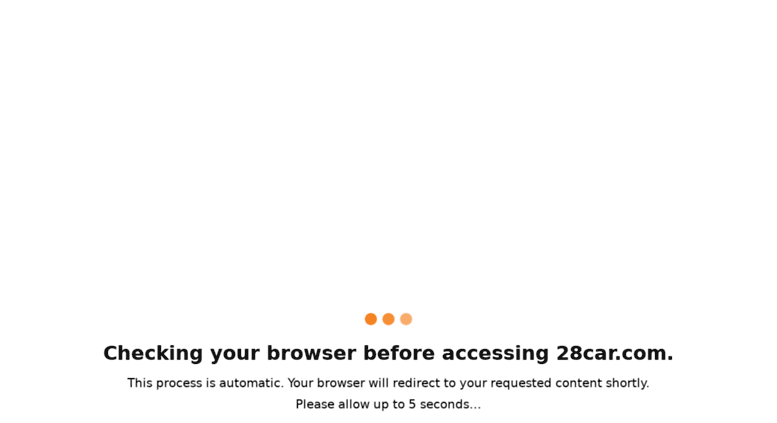This image captures a snapshot of a browser security check page for the website 28car.com. The page is presented without any external borders and features a dark grey square backdrop. Dominating the center of the image is a primary white background. Towards the lower center of this white section, three horizontally aligned dots convey a loading sequence. Each dot varies in color intensity: the left dot is a deep orange, the middle dot a brighter orange, and the right dot a peachy lighter orange. Beneath these animated ellipses, a clear message in black text reads: "Checking your browser before accessing 28car.com". Following this, a smaller black font explains the process: "This process is automatic. Your browser will redirect you to your requested content shortly. Please allow up to five seconds." The page implies that it is verifying the browser's integrity before granting access, with the animated dots likely indicating real-time progress. The domain 28car.com suggests a possible connection to automotive information or services, although no detailed specifics about the website's content are provided in the snapshot.